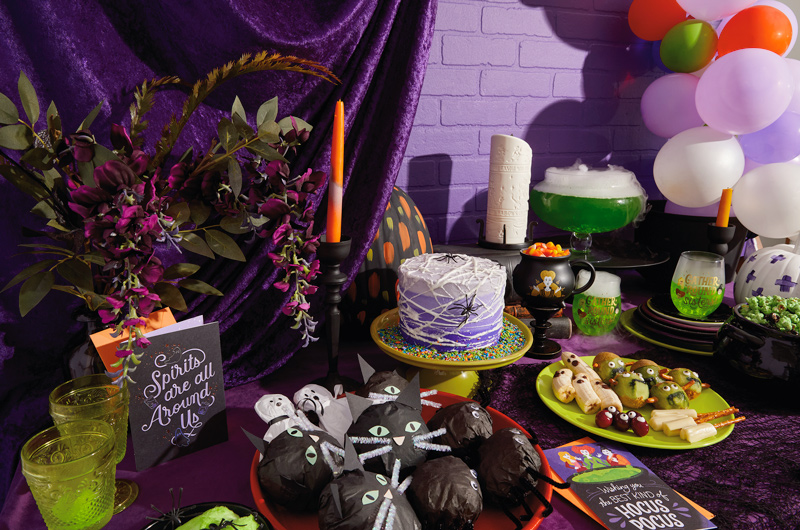The image depicts a vibrant table set up for a Halloween party, adorned in festive decorations. Dominating the scene is a Halloween-themed cake on a green cake stand, intricately decorated with purple and white icing and topped with black spiders. Surrounding the cake are various spooky treats, including bananas, grapes, and kiwis with adorable faces, and pretzel sticks creatively presented to resemble scary figures. The table also features a bowl of bubbling green liquid emitting smoke, contributing to the eerie atmosphere. Additional confections include green popcorn and a variety of colorful goodies.

Decorative elements enhance the festive mood, with a purple drape alongside a matching purple brick wall serving as the backdrop. The table is accented with an array of balloons in orange, green, purple, pink, and white colors, along with orange candles and black candle holders. Scattered among the treats are paper cut-outs of cats and ghosts, and a card with the phrase "Wishing you the best kind of hocus-pocus,” adding a charming touch to the display. A small floral arrangement with purple leaves further embellishes the scene, creating a spooky yet delightful setting suitable for a children’s Halloween party.